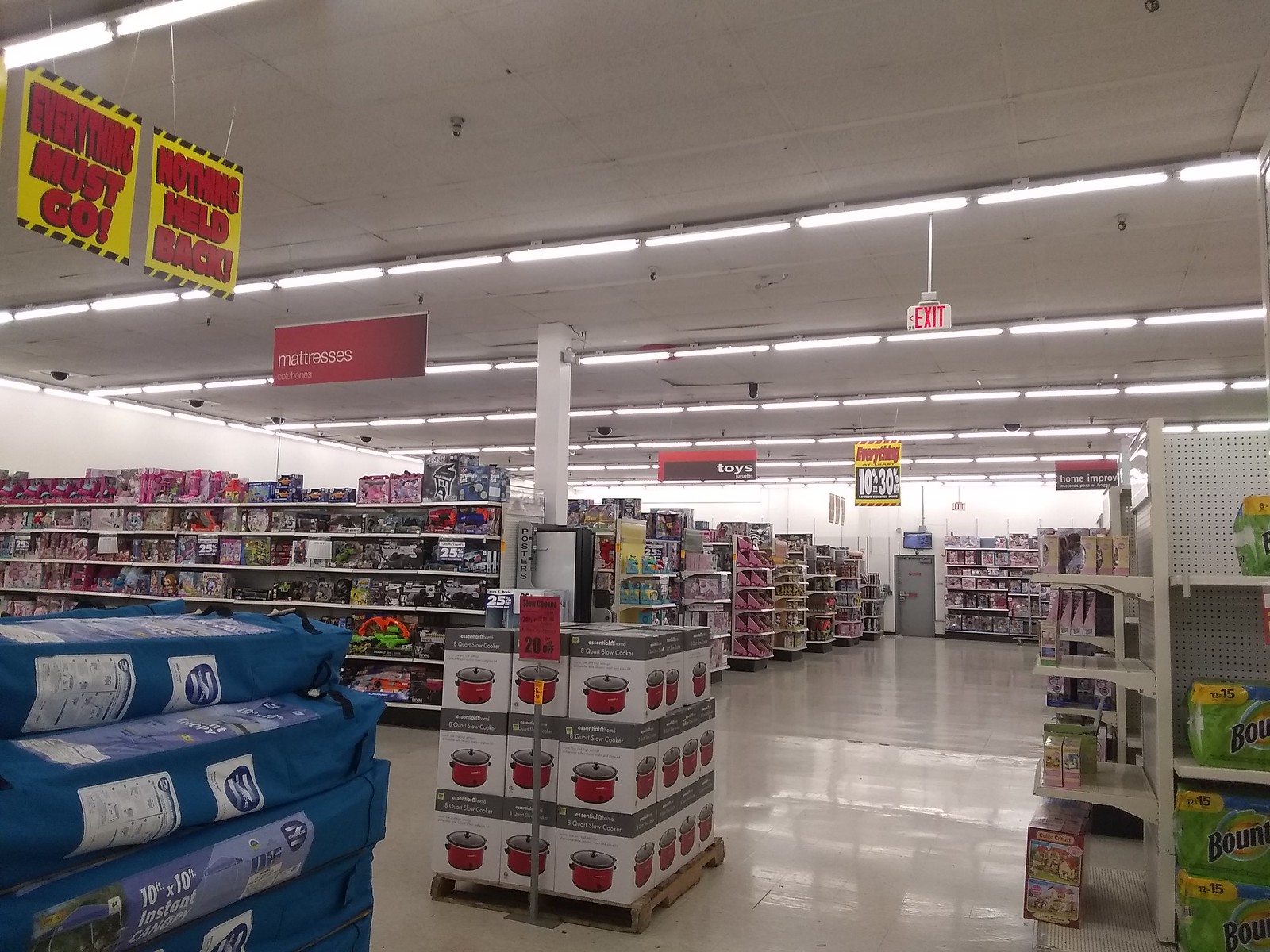The photograph, wider than it is tall, captures the interior of a bustling grocery supermarket. The roof, occupying approximately the upper third of the image, spans across the shot, while the rest of the frame is filled with an intricate array of grocery aisles and shelving units. Clearly visible are eight horizontal aisles stretching from the viewer's perspective towards the far wall. 

On the far left, a blue canopy signifies the camping gear section, marking the beginning of the shopping space. Adjacent to it in the same aisle, vivid pink dolls and a selection of colorful children's toys, including toy musical instruments or water guns, are prominently displayed. 

The center of the image showcases various crockpots and slow cookers, neatly arranged for shoppers interested in kitchen appliances. Towards the right, an aisle brims with household essentials like Bounty paper towels and an assortment of cereals, catering to everyday needs.

The other aisles, though less discernible, seem to be dedicated to toys and home improvement items, hinting at the diverse range of products available in this supermarket. The layout and organization emphasize convenience for shoppers, with clearly defined sections for specific types of goods.